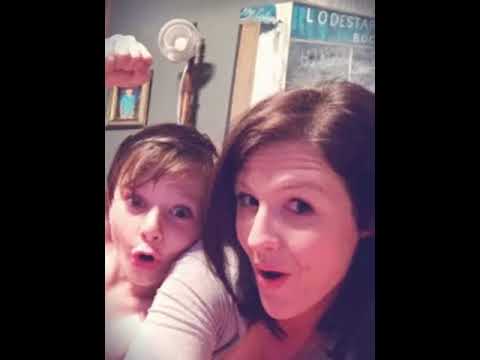In the image, a woman and a child are taking a playful selfie, likely intended for social media. The woman, presumed to be the mother, is on the right side of the image with short brown hair that curves under her chin. She is making an 'O' face and looking at the camera from the corner of her eyes, dressed in a gray sweatshirt. Beside her, on the left, is the child, possibly around 10 or 11 years old. The child, shirtless with wet blonde hair, appears to have just come from the pool, bath, or shower and is enthusiastically posing with a fist raised above his head, also mimicking an 'O' face. The two are centered in the photo. In the background, there is a white fan mounted on a brown post on the wall with a white cord hanging down, and a picture frame is visible in the top left. The colors featured in the photo include tan, gray, brown, blue, and green. The scene suggests an indoor setting, likely during the middle of the day.